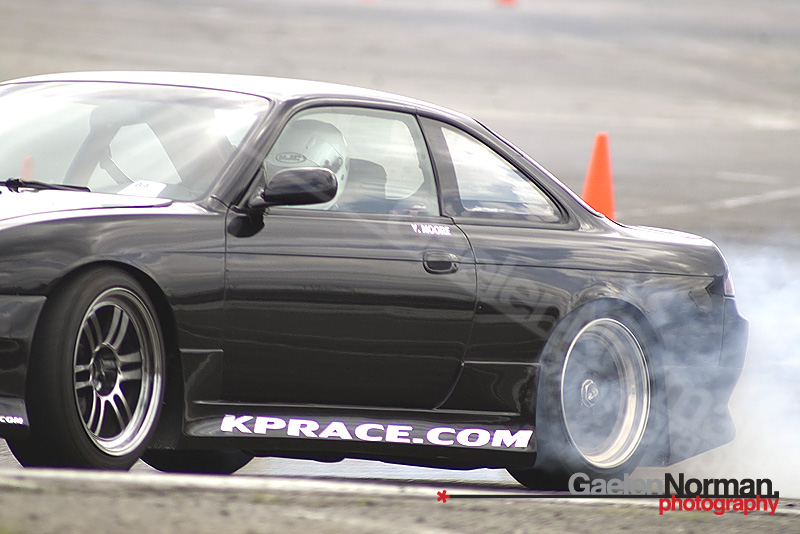This detailed outdoor photograph, captured by Gaelip Norman Photography, depicts a sleek, black two-door sedan race car in motion on a racetrack. The car, seen facing from right to left, is burning out, producing a thick cloud of smoke from its rear tire indicating a high-speed maneuver. The driver, whose face is obscured by the side view mirror, is wearing a white helmet, suggesting professional racing. Notably, the car features the text "kprace.com" in white print with a purple outline along the fender underneath the door. An orange traffic cone is visible in the background, enhancing the racetrack setting. The image is meticulously watermarked, from the upper left to the lower right in light transparent gray lettering, with "Galen Norman Photography" and an additional signature in the lower right corner: "Galen Norman" in black, with "Photography" below in red, annotated with a red asterisk and an underlining black line.